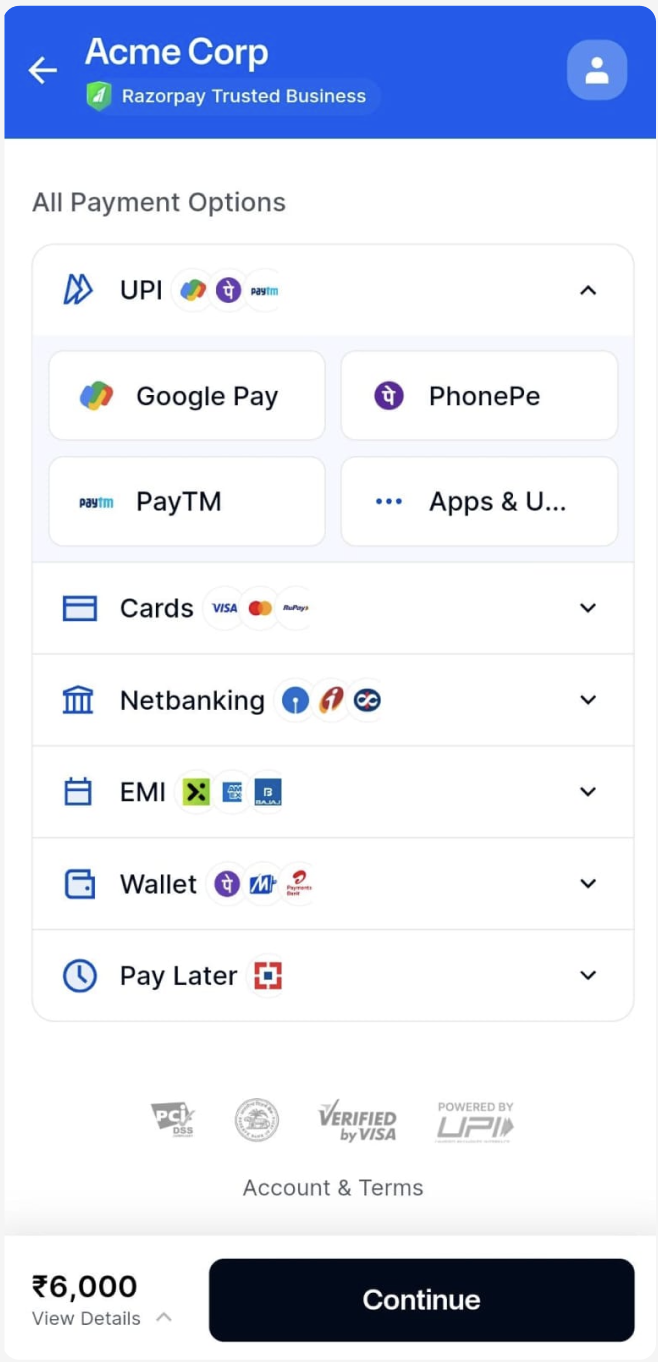A screen capture from a mobile phone displaying the payment options for Acme Corp. At the top of the screen, the Acme Corp logo, represented by the letter "A," is prominently featured. Below the logo, the text "Razorpay Trusted Business" is accompanied by a shield icon, emphasizing security. A variety of payment methods are detailed on the screen:

- **Cards**: Options include Visa, MasterCard, RuPay, and more.
- **UPI**: Users can pay with an installed app or choose from alternatives like Google Pay, PhonePe, Paytm, and others.
- **NetBanking**: A comprehensive list of all Indian banks is provided.
- **Wallet**: Payment options include PhonePe and others.
- **EMI**: Flexibility with EMI via cards, OneCard, and additional choices.

An account balance is shown with an upward-pointing arrow, highlighting 6,000 units of an unspecified currency. A prominent blue button labeled "Pay Now" invites users to complete their transactions. This screen appears to be part of a payment interface, offering a broad range of options for users to pay Acme Corp or for Acme Corp to facilitate payments, ensuring versatility and convenience for all transactions.